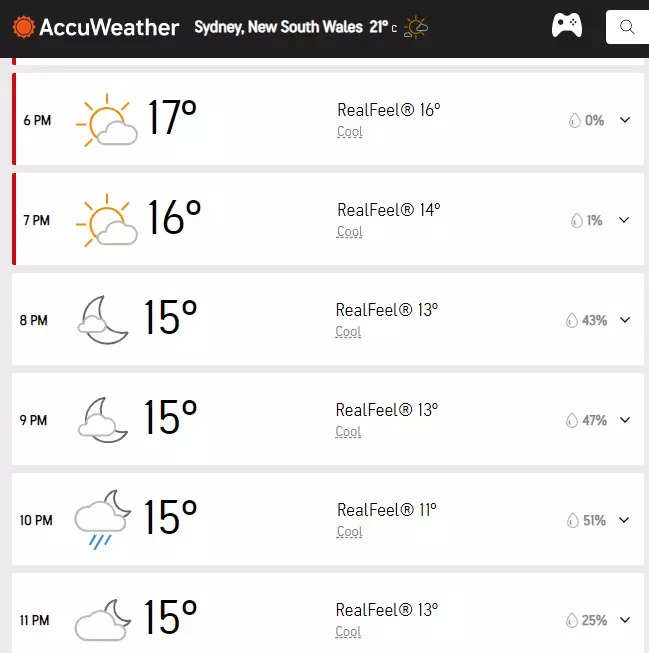This portrait-oriented screenshot captures the display of a weather app, specifically showing a detailed hourly weather forecast for Sydney, New South Wales. The top of the screen features a horizontal black bar with "AccuWeather" written in white text next to a red or orange sun icon. Alongside are a video game controller icon and a search bar.

Below the top bar, the weather forecast is broken down by hour, displayed in six vertically stacked white rectangular boxes with black text. Each box presents icons representing different weather conditions and specific hourly details, from 6 p.m. to 11 p.m.

The highlighted hours, 6 p.m. and 7 p.m., feature red vertical indicators on their left side. The weather icons depict various scenarios such as a sun partly obscured by a cloud, a moon with varying amounts of cloud cover, and a moon with rain clouds.

Temperatures begin at 17 degrees Celsius at 6 p.m., decreasing to 15 degrees Celsius by 11 p.m. Additionally, the "RealFeel" temperatures range from 16 degrees at the start to 13 degrees at the end of the forecast period. On the far right, the percentage likelihood of rain is displayed with accompanying drop-down arrows, starting at 0% and increasing to 25% by 11 p.m. The visually appealing format provides a comprehensive and easy-to-understand snapshot of the anticipated weather conditions for the evening.